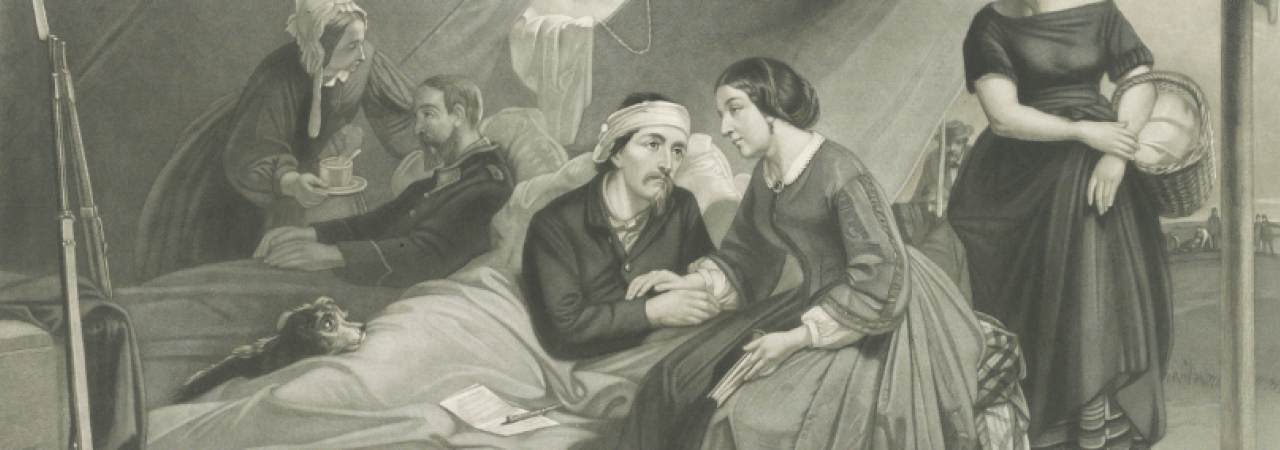The detailed black and white illustration captures a serene yet poignant 17th to 18th-century scene within a tent-like hospital setting, likely from a wartime period. At the forefront, two wounded military men lie in two separate beds. One man, dressed in pajamas with a bandage wrapped around his head, engages in a heartfelt conversation with a lady sitting beside him. This woman, adorned in a long, poofy-sleeved dress with a gathered skirt, exudes care and tenderness. Resting its head on the man's leg is a solemn dog, embodying the gravity of the scene. 

The second bed cradles a bearded man in a military uniform. A woman, similarly dressed in the period's attire, comforts him while holding what seems to be a cup or mug with a saucer. Surrounding these central figures are several background individuals, including a woman with a basket of white pillows and others who appear to be working, adding depth to the scene. The artwork intricately details the interactions and emotional undertones of a time steeped in historical significance and human compassion.